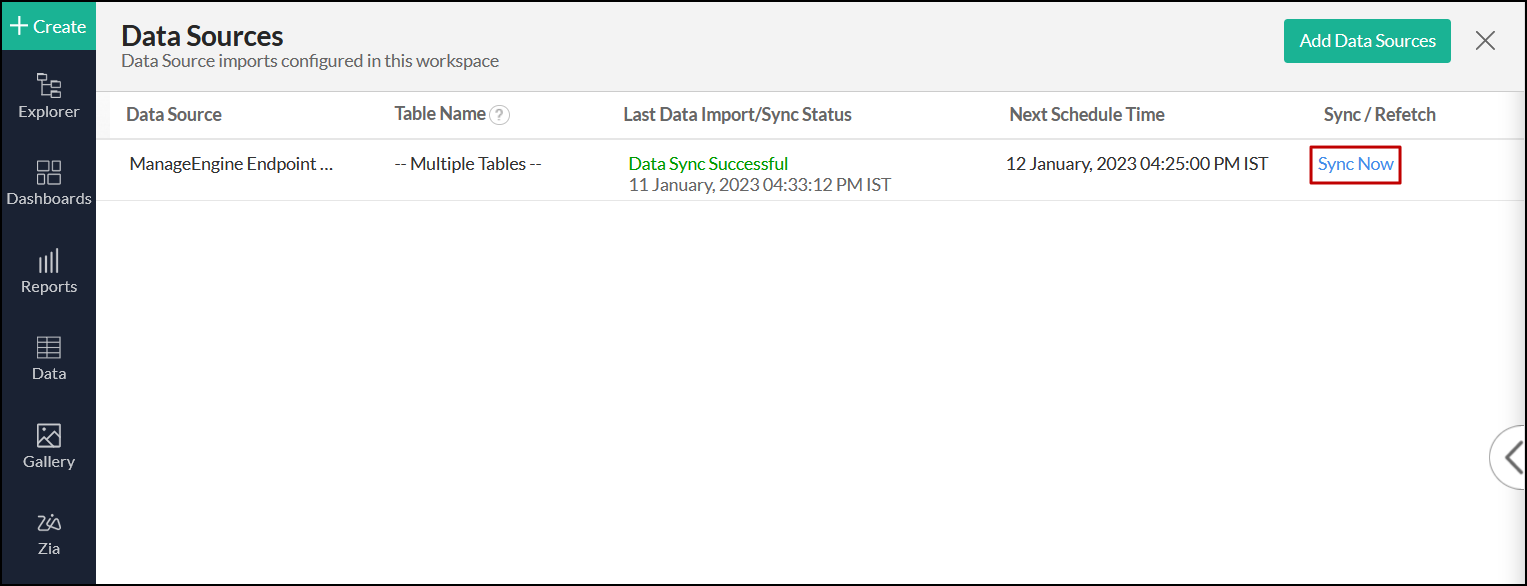This is a detailed screenshot capturing the backend interface of a website's management system. The page is structured with a prominent vertical sidebar on the left side of the screen. At the top of this sidebar, there is a horizontal menu with a green button labeled "Create," featuring a plus sign and the word "Create" in white text.

Beneath this top menu, the left sidebar presents six options, each accompanied by a relevant icon: Explorer, Dashboards, Reports, Data, Gallery, and another unspecified symbol. 

On the upper right side of the screen, there is a section labeled "Data Sources." Adjacent to this label, on the far right, is another green button that says "Add Data Sources" in white text. The interface is designed to manage various columns and data inputs, suggesting robust functionality for data organization and reporting.